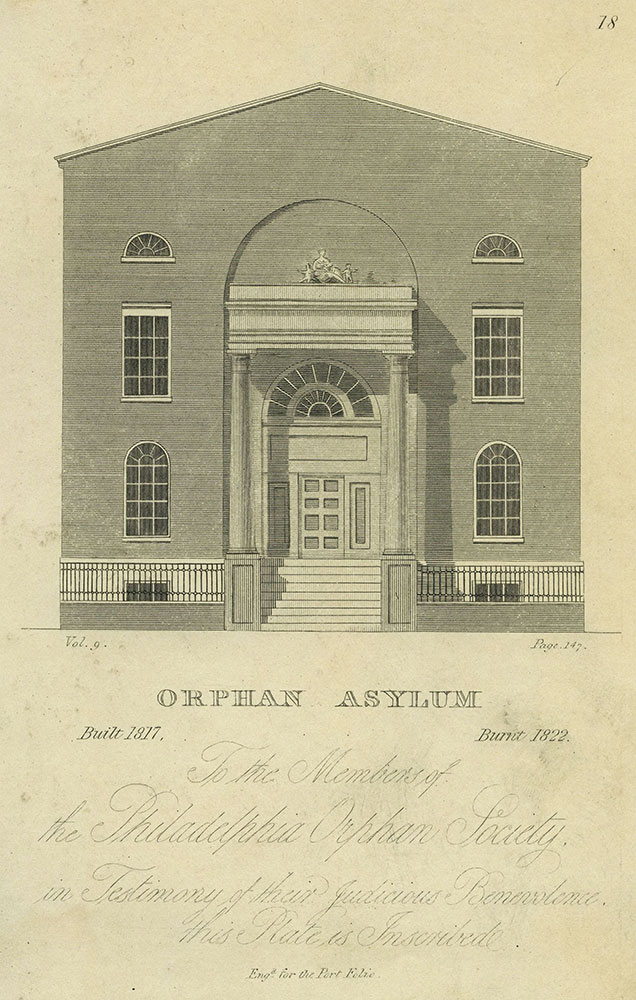The image appears to be a black and white scan from an old book or poster, featuring an illustration of an imposing, boxy building labeled "Orphan Asylum." The building, constructed in 1817 and burned in 1822, is gray and detailed with ornate windows and a set of white stairs leading up to a covered front door, supported by two large pillars. At the top of the image, there's a page number "18" in the top right corner. The background shows signs of age, with a tan hue and black spots, resembling old paper. Below the illustration, there’s a series of lines in fine, cursive text that are difficult to read, but it includes a dedication to the members of the Philadelphia Orphan Facility.